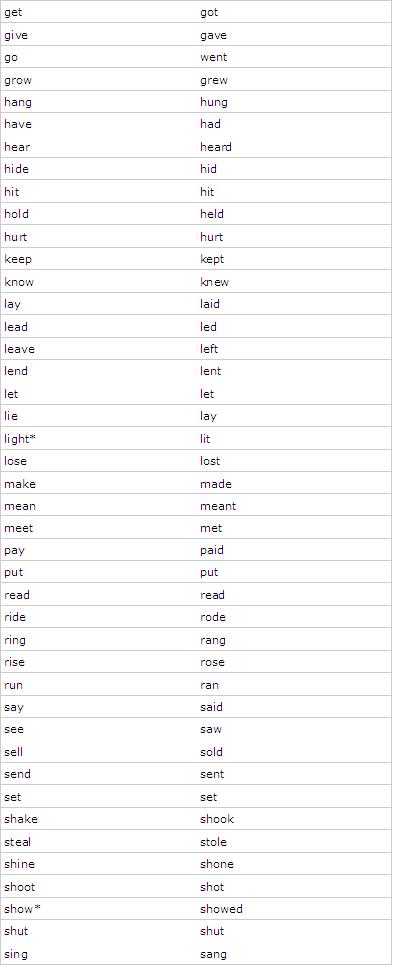The image depicts a neatly organized table with two columns showcasing individual words arranged in alphabetical order. The left column lists verbs in their present tense forms, while the right column displays the corresponding past tense forms. Each row pairs a present tense verb with its past tense counterpart, reading across from left to right. For example, the first row pairs "Get" with "Got". Subsequent rows include pairs such as "Give" with "Gave", "Go" with "Went", "Grow" with "Grew", "Hang" with "Hung", and so on. The table continues with pairs like "Have, Had", "Hear, Heard", "Hide, Hid", "Hit, Hit", "Hold, Held", "Hurt, Hurt", "Keep, Kept", "Know, Knew", "Lay, Laid", "Lead, Led", "Leave, Left", "Lend, Lent", "Let, Let", "Lie, Lay", "Light, Lit", "Lose, Lost", "Make, Made", "Mean, Meant", "Meet, Met", "Pay, Paid", "Put, Put", "Read, Read", "Ride, Rode", "Ring, Rang", "Rise, Rose", and it continues further in a similar format. This structured presentation makes it easy to compare the tense variations of each verb, serving as a useful reference for understanding verb conjugation.